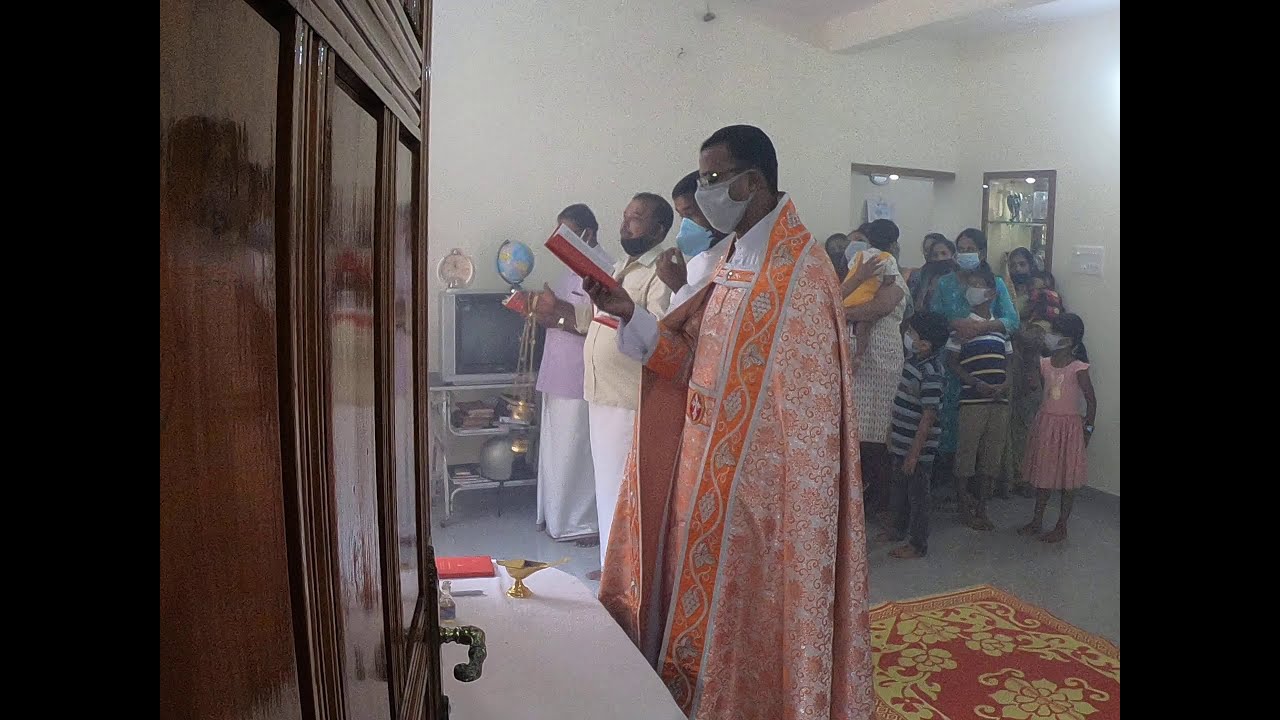The photograph captures an indoor religious gathering within what appears to be a makeshift place of worship that resembles a regular room rather than a traditional church. The setting features plain white plaster walls and a simple atmosphere. At the center of the scene, a man, presumably the priest, stands out in elaborate orange and white robes adorned with intricate, likely Indian, symbols. This robed figure, who also wears glasses and a COVID-type face mask, holds a red book in his hands.

He is accompanied by three other men standing in a row, all engaged in some form of reading or chanting from their books, facing towards the left side of the image. Situated near them is a small white table that might hold a communion vessel or other religious items. Behind this group is a crowd of observers, predominantly Indian, many of whom are middle-aged women with children. These onlookers are also wearing face masks, indicating the precautions being observed during the event.

The room features a red and yellow rug on the floor, adding to the simple yet vibrant setting. In the distance, a television can be seen, subtly blending into the background, while on the left side, there's a large wooden cabinet structure. Light filters into the room from an unseen source, casting a serene ambience over this intimate gathering focused on prayer and community.